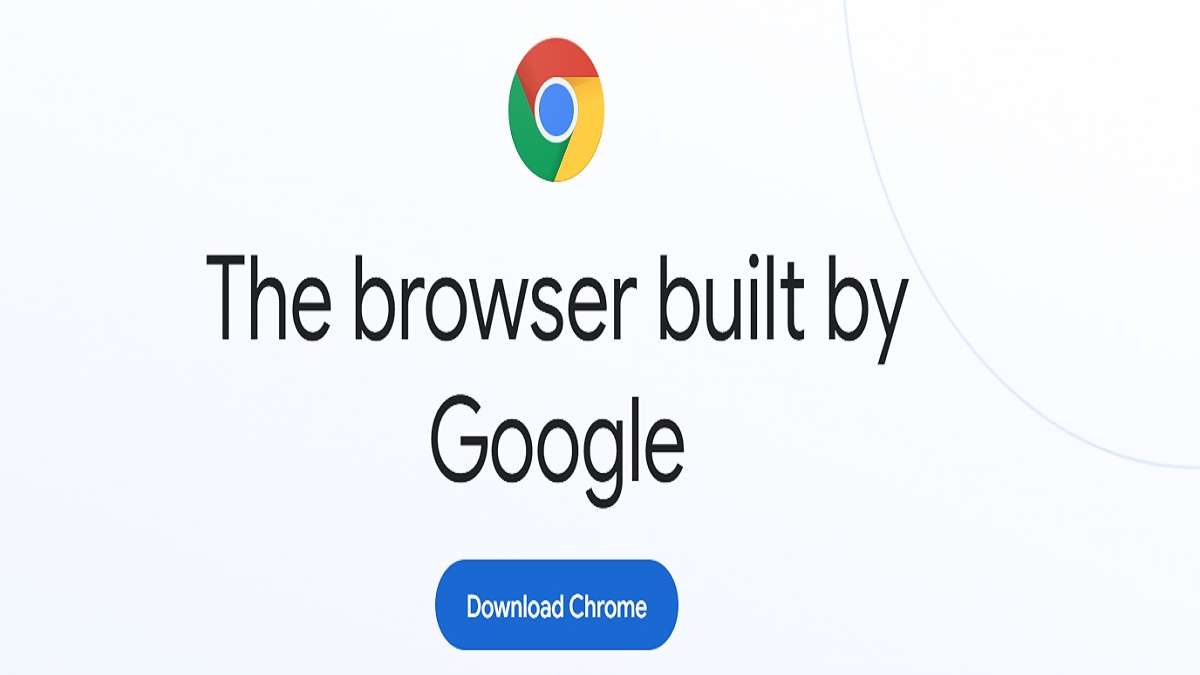The image is a minimalistic advertisement for the Chrome browser, exuding simplicity and clarity. At the top, it prominently features the recognizable Chrome logo, a circle segmented into a red upper section, a green lower-left section, a yellow lower-right section, and a central blue circle. Directly beneath the logo, large, bold text reads "The browser built by" on one line, with "Google" on the subsequent line, emphasizing the brand's credibility. Further down, a blue, clickable button stands out, bearing the text "Download Chrome" in white, inviting users to engage. The overall design is stark and uncluttered, featuring no additional visual elements, focusing solely on the essential information and call to action.